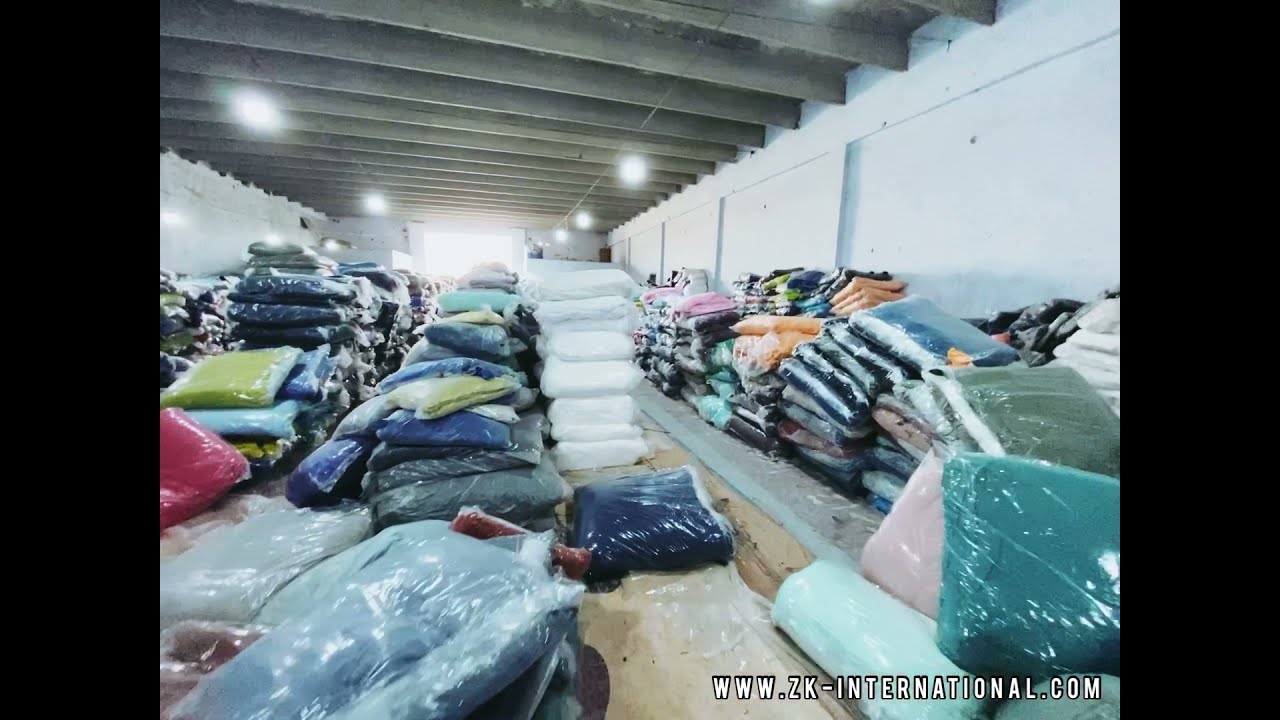This image showcases the interior of a long warehouse or storage area filled with a variety of fabric products, predominantly blankets in assorted dark colors like blue, green, and orange. These fabric items are individually wrapped in plastic and stacked in piles throughout the space. The warehouse has white walls and an unfinished loft-style ceiling, with exposed wooden support beams. Strung across these beams are lines of fluorescent lights, adding illumination to the scene. To the center-left of the image, a large open entrance resembling a garage door allows natural light to seep into the room. At the bottom right corner of the image, the text "www.zk-international.com" is visible, with black borders on the left and right edges of the image.